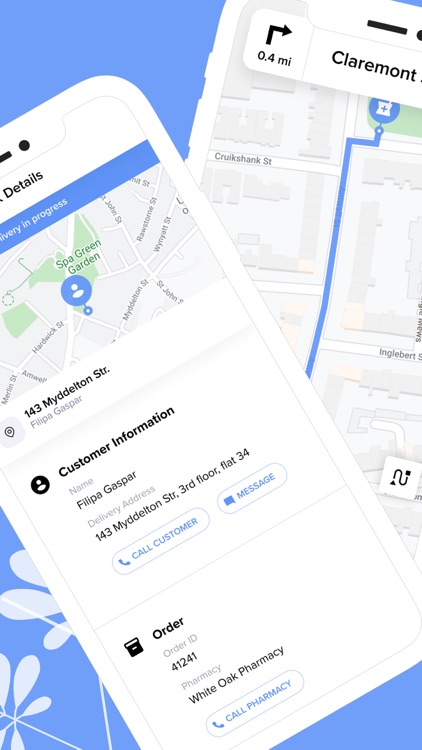The image presented is a vertically oriented artist's representation, roughly twice to two and a half times as tall as it is wide, featuring two overlapping white cell phones. The main focus is on the top cell phone, which is angled towards the 11 o'clock position and occupies the majority of the frame. This cell phone partially obscures another beneath it, which is angled around the 12:30 position. The bottom left third of the underlying phone is cut off by the edges of the image.

The screens of both cell phones display different map-related content. The lower phone presents a map application, likely Google Maps, showcasing a blue route traversing a road. The upper phone features a smaller map occupying the top quarter to third of the screen. Below this map is text detailing delivery information. It lists an address, "143 Middleton Street," followed by "Customer Information" and the customer's name, "Philippa Gaspar." Additional details include the delivery address repeatedly noted as "143..." indicating the purposes of navigation and delivery coordination.